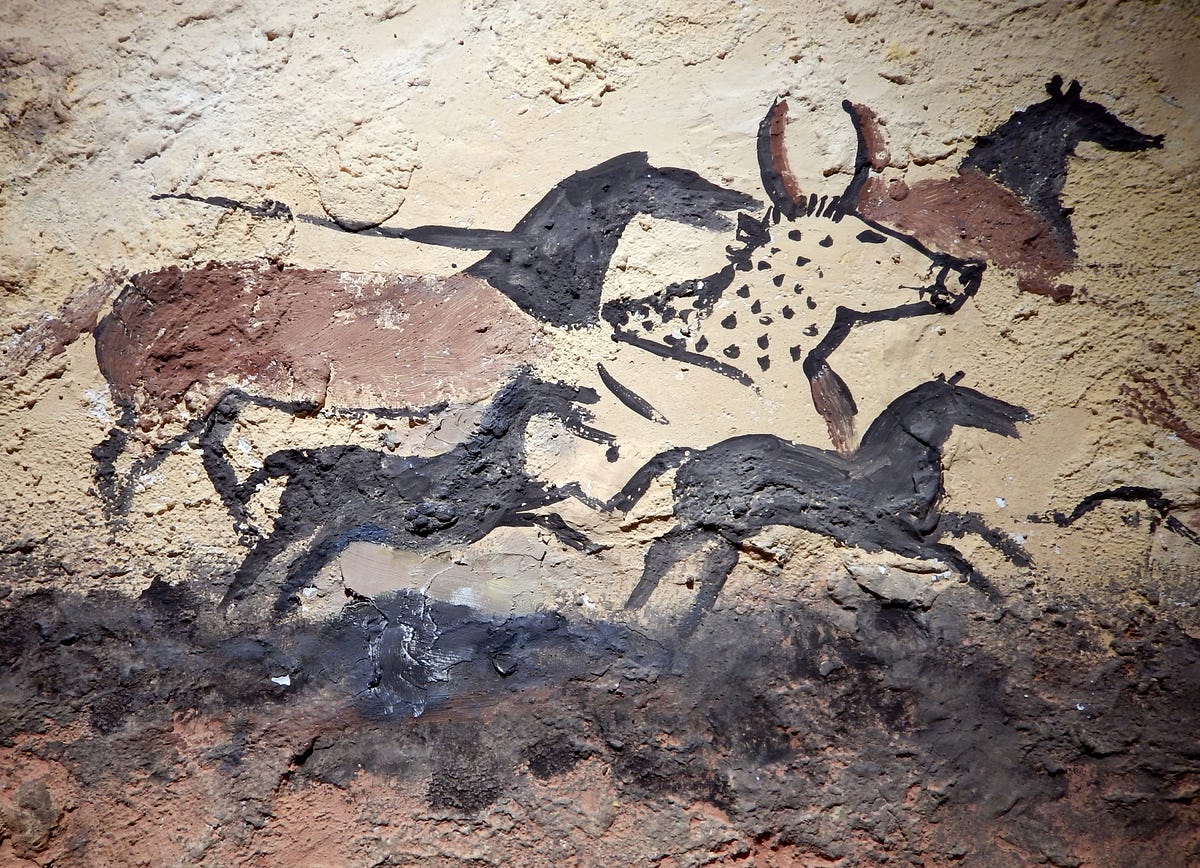The image is a color photograph of a cave painting depicted on a rough, brown, and scraped-up stone wall. The upper three-quarters of the background shift to a light beige color, while the bottom fourth transitions into darker blacks and browns, featuring scattered black streaks as if painted with fingers. The central focus is a rudimentary painting using brown and black pigments, showcasing a series of five animals, primarily horses. Two small black horses appear at the bottom, galloping energetically. In the middle, there is a brown horse with a black head and a horizontal black line emerging from its neck, partially cut off. To the upper right, another brown horse with a black head is depicted. Additionally, there is a white spotted, deer-like animal's head with brown antlers just right of the center. The overall composition conveys a dynamic sense of motion among the animals.